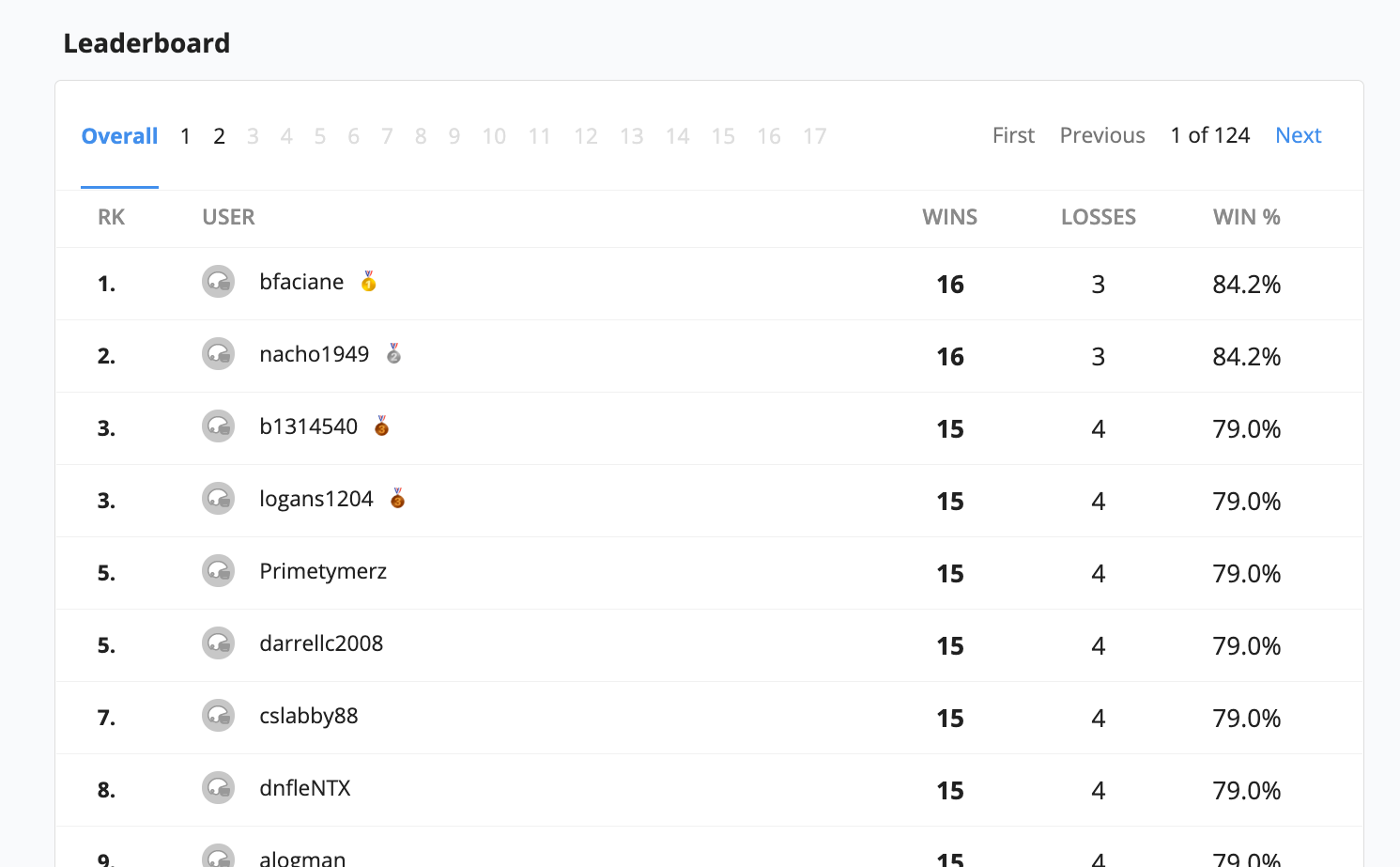Screenshot of a Leaderboard: This image captures a screenshot of an unidentified game's leaderboard, showcasing the overall rankings of players. The leaderboard spans 124 pages, but the visible portion highlights the top nine players. 

At the top, the player B. Fakane holds the first position with a gold medal, recording 16 wins, 3 losses, and an 84.2% win ratio. Nacho1949 ranks second, also with 16 wins and 3 losses. The third position is tied between two players, each boasting 15 wins and 4 losses, a win ratio that extends consistently from ranks three to nine. This close ranking signifies a very competitive standing among the top players, all sharing similar records. Below these top nine, the remaining rankings are not visible.